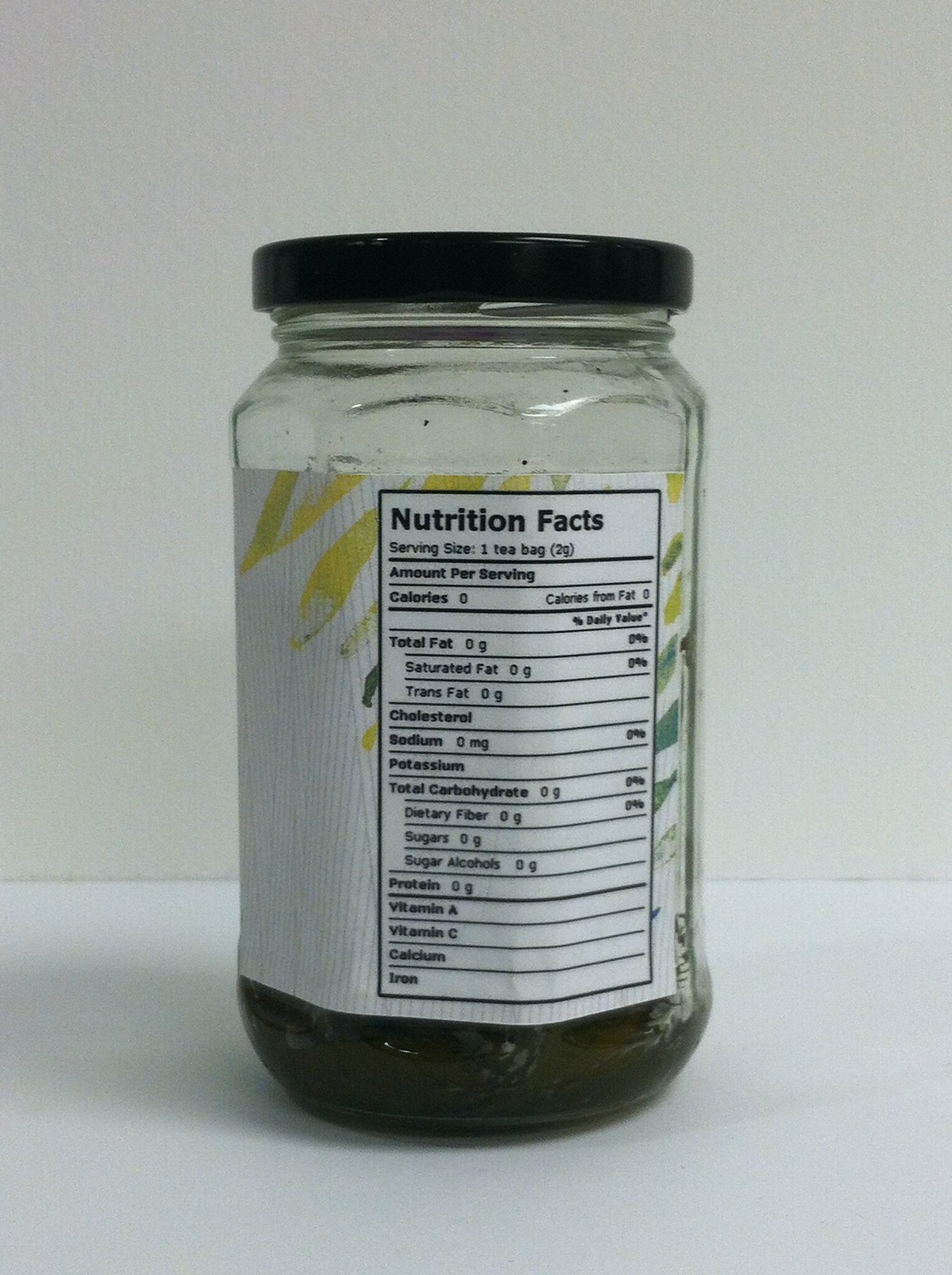This color photograph showcases a glass jar with a black or possibly very dark lid placed on a light gray countertop. The backdrop is a similarly gray-tinted wall. The jar, which appears to contain food, is oriented with its back facing the camera, displaying a label that covers the majority of the jar. At the bottom of the jar, a dark, greenish substance is visible, hinting at its contents. The label prominently features a "Nutrition Facts" heading, but the text is too small to be legibly read in the image.